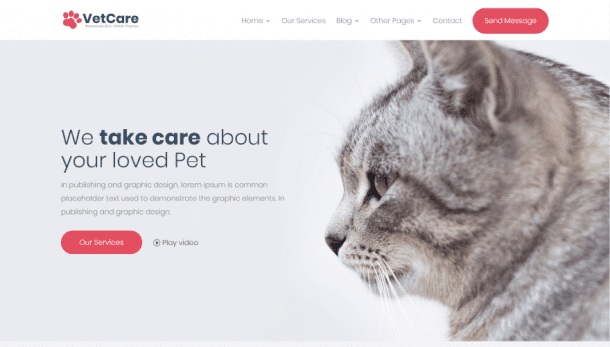In this image, we see a clean, solid white background with a gray box positioned in the upper left corner. This box features bold black text reading "Vet Care," accompanied by a red animal paw print to its left. To the right of this, in light gray text, are navigational links labeled "Home," "Our Services," "Blog," "Other Pages," and "Contact." Additionally, there is a red box containing the text "Send Image."

Beneath this section, there is an image showcasing the left profile of a gray and black tabby cat's head, with the cat facing westward. A bold black message below the tabby cat's image reads, "We take care of your loved pet." Following this statement is the placeholder text "Lorem ipsum," commonly used in publishing and graphic design to indicate where real content will eventually be placed.

Further down, there is a red box with white text labeled "Our Services," tying back to the navigation mentioned at the top, indicating a call-to-action for viewers interested in the veterinary services offered.